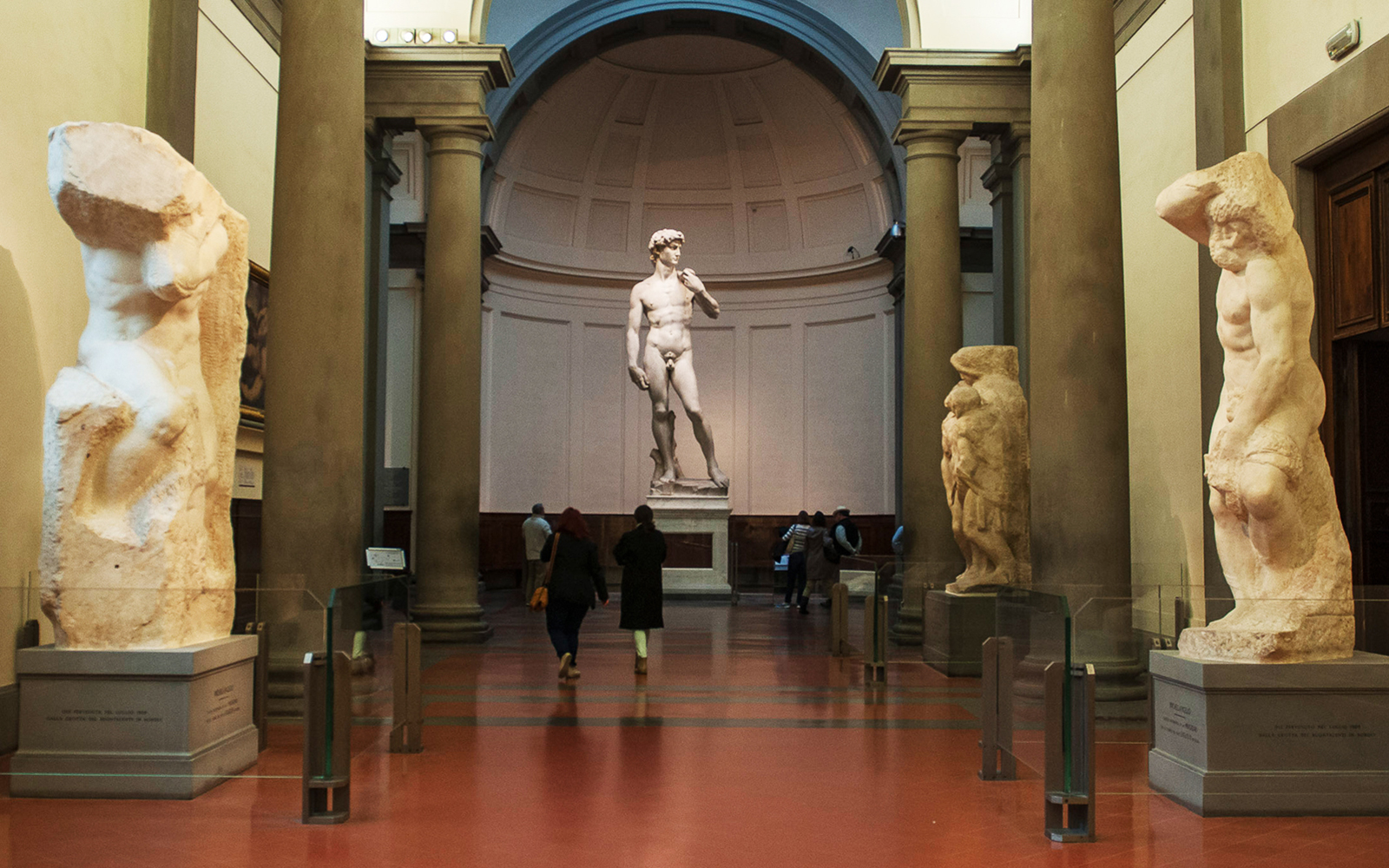The photograph captures the grand interior of a museum, showcasing a horizontally aligned room with a design reminiscent of a hallway. The floor is a medium cherry-brown tile with accent lines that guide the eye towards the central feature. Along the left and right sides, tall statues, each perched atop light-gray square pedestals adorned with black text, line the path. These statues are composed of light tan stone; one on the right depicts a shirtless man with a dynamic pose of one leg up and arms in varied positions. The statue on the left appears to be a human figure wrapped in stone, with its head visible.

Further down, the focal point is a domed ceiling in a light-brown stone housing an impressive marble statue of a naked man, possibly the statue of David, standing against the intricate backdrop. The statue, facing the camera but gazing to the left, stands on a pedestal centered in the domed alcove. Flanking the statue are colossal greenish-gray columns that add to the grandeur of the space.

The scene is animated by museum visitors, including a couple of women in black jackets positioned in the middle of the hall, with more individuals scattered, looking up at the central statue, enhancing the dynamic and vibrant atmosphere of the museum.